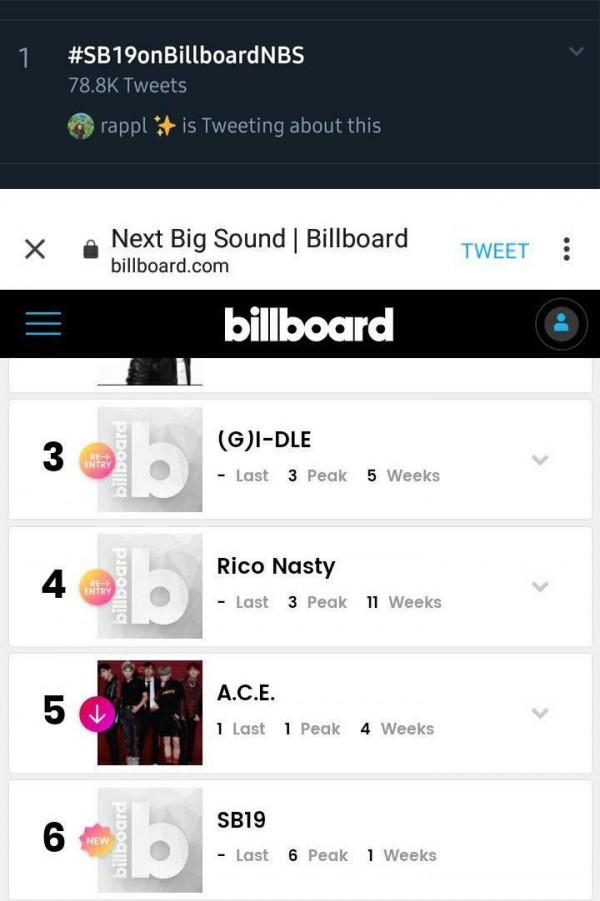A detailed image description of a billboard depicts a website interface with various elements related to trending topics and chart rankings. At the top, the website prominently displays the text "#SB19 on Billboard MBS," with a count of 78,800 tweets listed below it. To the left side, the number "1" is visible, indicating a top ranking or position.

Beneath the tweet count, there is a section labeled "RAPPL," accompanied by a user profile picture. Adjacent to this label, the words "tweeting about this" appear. Below this, on a white background with black text, the inscription "Next Big Sound" is evident. Directly underneath, the URL "billboard.com" can be seen.

To the right of these elements, the word "tweet" is highlighted in blue text. Further down, another section with a black background and white text reads "billboard," with a user profile picture identified as "JRick" located to its right. 

In the lower section, only rankings 3 through 6 of the Billboard chart are partially visible. The second ranking's number is not fully shown, only the bottom half of the artwork is noticeable. The third ranking is marked as a "re-entry," displaying a blue and orange-reddish circle atop the Billboard "B" logo. Adjacent to this, it reads "(G)I-DLE," with its last week's ranking at 3 and a peak position maintained for 5 weeks. There is also a dropdown box for additional information.

Following this, the fourth spot is held by Rico Nasty, who was previously at 3 for 11 weeks. Ranking at number 5 is "Ace," which has dropped a spot from last week's number 1, where it peaked for 4 weeks. Lastly, number 6 is occupied by SB19, consistent with last week's ranking, having peaked at that position for 1 week.